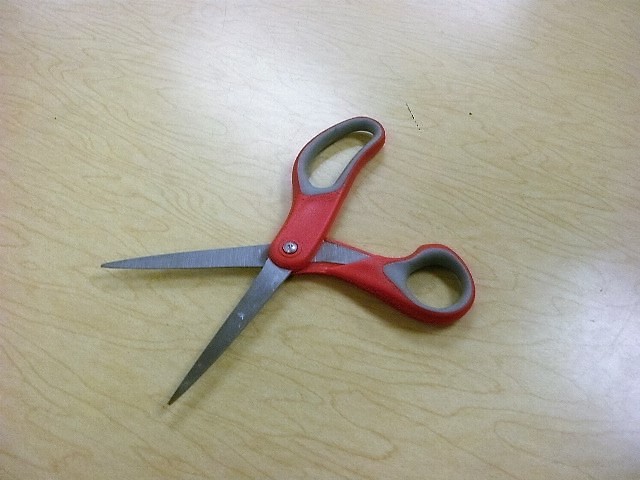The color photograph captures a detailed top-down view of a pair of scissors laid open on a tabletop. The tabletop features a light, yellowish wooden color with visible grain, giving it a manufactured wood appearance. It appears somewhat dirty, with visible marks and scuffs, illuminated from above with light reflecting on the right-hand side. Dominating the center of the image, the scissors are completely open in a cross-like position. The handles are predominantly red with gray finger cutouts, suggesting a mix of plastic and metal elements. The blades are dark gray and one handle hole is designed to be round while the other is elongated for the thumb. The scissor tips point towards the lower left corner, with a silver screw at the junction holding the two halves together.